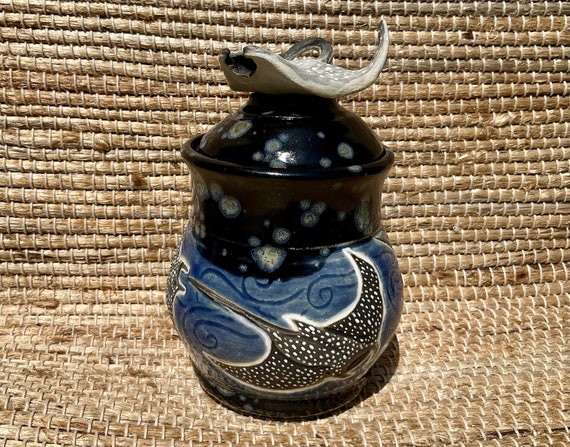The image features a carefully crafted piece of pottery, resembling a jar or vase, which is resting on a woven thatched mat made of brown reed-like material with white thread accents. The pottery itself showcases a harmonious blend of blue tones—ranging from dark to light—symbolizing the ocean. The lower part of the jar displays a vivid depiction of a black stingray with white polka dots, swimming across the blue background with swirling designs that evoke the movement of water. The upper part transitions into a darker blue, adorned with small speckles, possibly representing starlight or bubbles. Atop the jar, the lid features a sculpted handle shaped like a stylized stingray, integrating seamlessly with the oceanic theme of the piece.